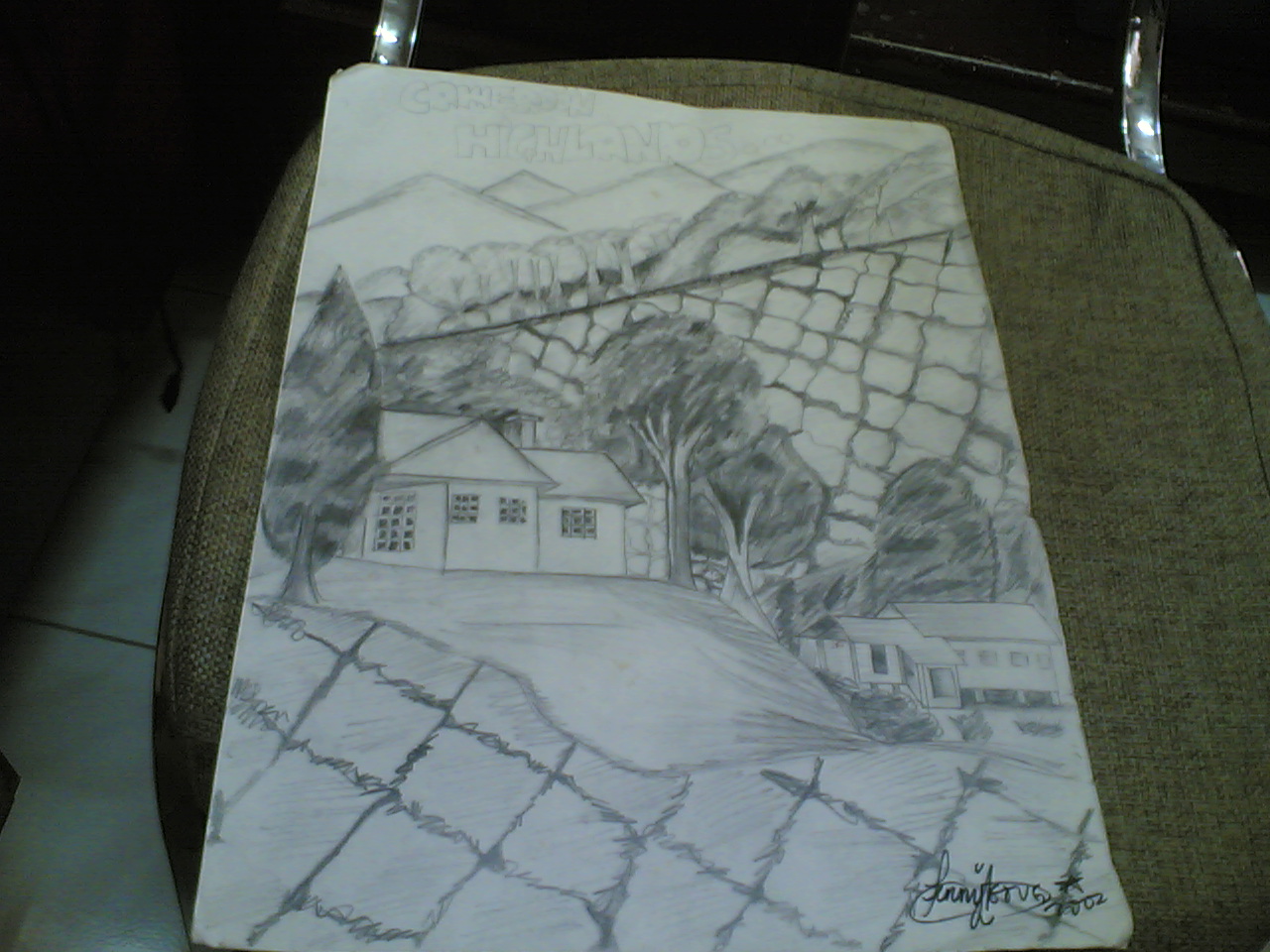This descriptive caption combines the details provided by all three individuals, placing emphasis on the common elements and specifics:

This is a detailed pencil sketch from 2002, signed by the author in the lower right-hand corner. The sketch features a rural landscape with two houses amidst a hillside setting. The main house sits on a hill, with a rolling yard extending downwards, and features a chimney, three front windows, and a driveway. Adjacent to it, on the right, is a smaller, farm-style house with a porch. The scene is adorned with various trees and bushes, including a large tree resembling a leaf with a pointed top and a rounded-top tree. Behind the houses, a diagonal hill dotted with trees rises to the right, leading to sharp-peaked mountains in the far background. A fence, depicted with scribbly lines forming squares, separates the houses from the backdrop of hills and woods. Faint text in the background includes the word "highlands." The drawing is placed on a green-cushioned kitchen chair, framed in silver or aluminum, with a white tile floor visible at the side.